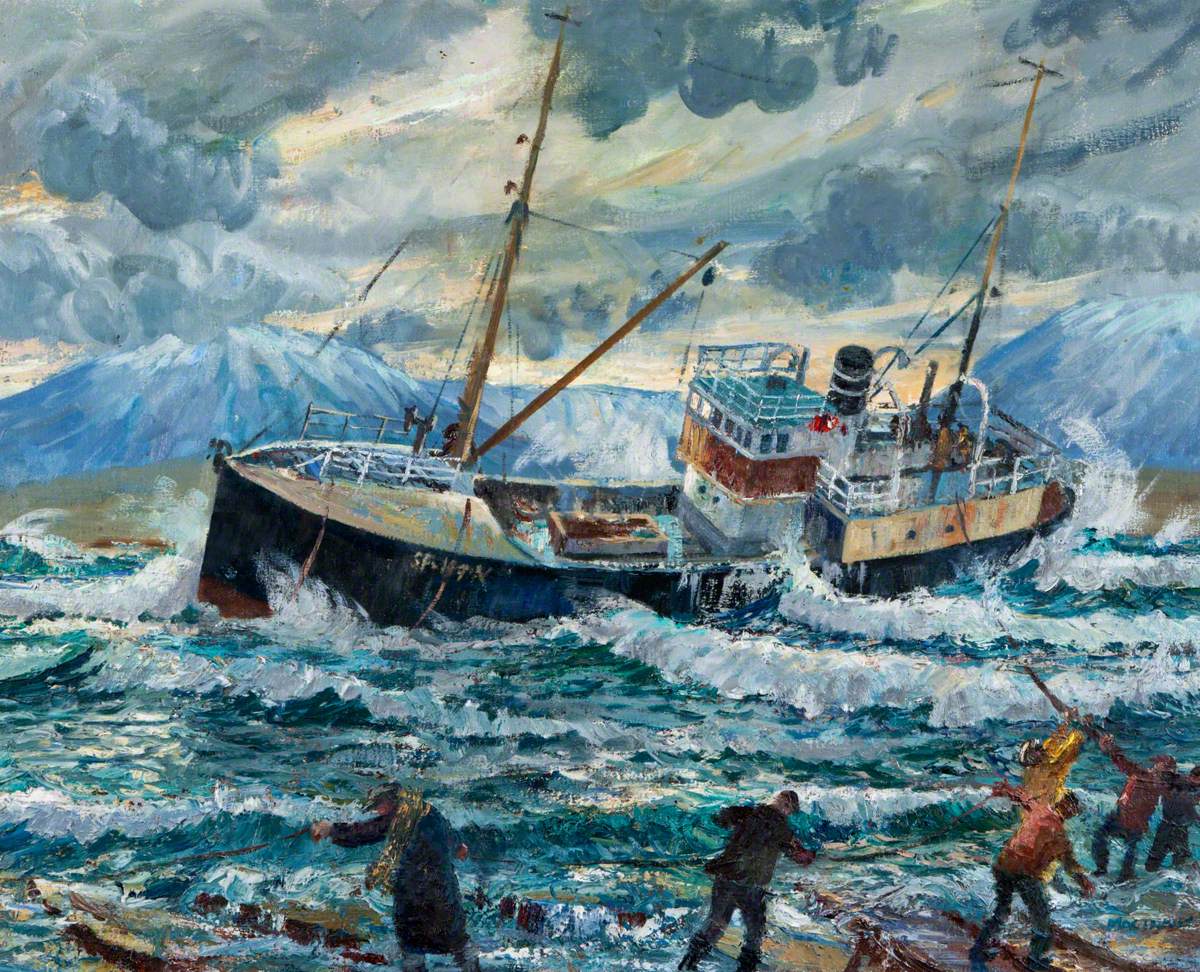This detailed painting captures the dramatic scene of a large fishing vessel caught in a violent ocean storm. The turbulent waves are intricately depicted with various textures and a captivating color palette of blues, grays, and whites, emphasizing the ferocity of the sea. The ship is precariously tilted on its side, with its blue base partially submerged in the frothy waves, and its poles and upper deck dangerously exposed to the elements. In the midst of this chaos, five men are seen standing on rocky terrain near the shore. One man in a yellow jacket clings to a piece of rope, while another in a red jacket tries to pull the rope, possibly attempting to rescue the ship or assist those still on board. The mountainous backdrop and ominous rain clouds add to the painting's intense atmosphere, portraying the relentless power of nature versus human struggle.